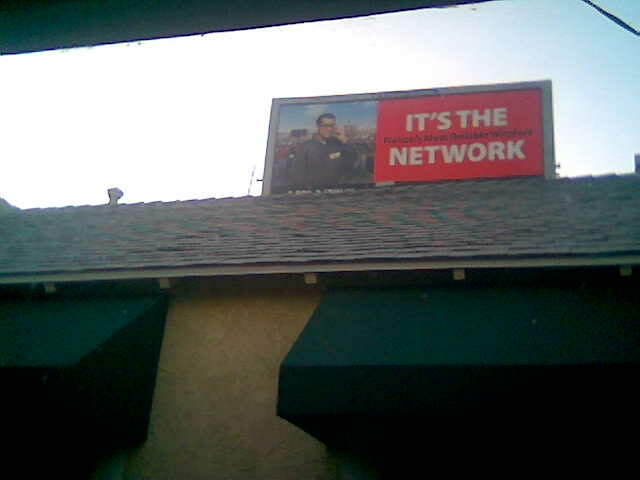The image is a low-resolution, square photograph that appears blurry and fuzzy. Despite the poor quality, the scene is discernible. It depicts a sky transitioning from white on the left to light blue on the top right. Below the sky, a black-colored roof is partially visible, topped by a rectangular signboard. The signboard has white text on the right that reads "It's the network," though the exact wording may be a bit difficult to decipher due to the image's blurriness. Additionally, there is some black text that is not clearly readable. On the left side of the signboard, there is a faint, indistinct image of a man.